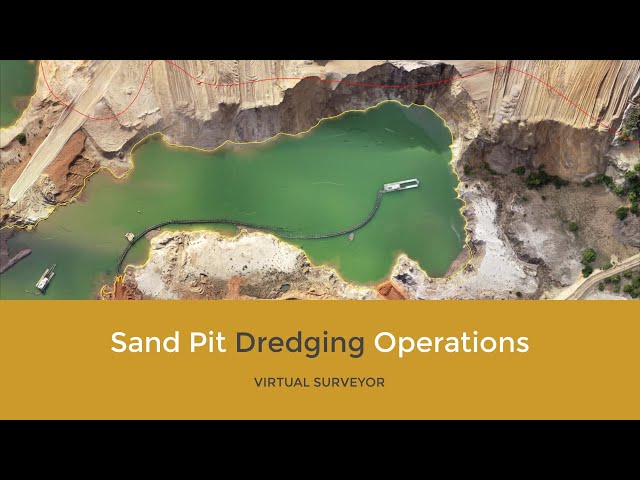The image depicts an overhead view of a sandpit with greenish-blue water at its center. This water body is bordered by sandy cliffs, giving the appearance of a deep excavation site. In the water, there are two small boats, each trailing a hose-like device, potentially used for dredging purposes. Surrounding the water, a faint red line outlines the section of land earmarked for dredging. The photograph itself spans the full width of the image, with black bars framing it at the top and bottom. At the bottom, a gold-colored banner with white text denotes "Sandpit," while black text in the middle reads "Dredging," and to the right, an additional white text states "Operations." Below this banner, there is smaller black text that reads "Virtual Surveyor," indicating that the image might be part of a survey report or an informational presentation about the dredging activities planned or currently happening in this sandpit area.